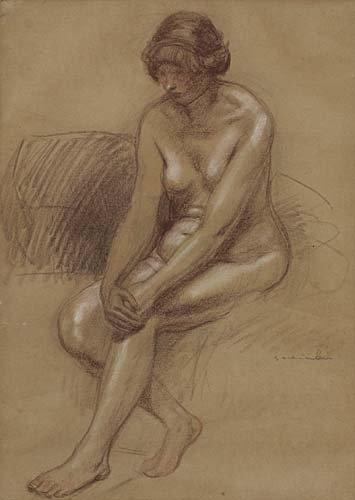This is a vertically oriented, portrait-style drawing by artist Steinlein in the Art Nouveau style. The image portrays a nude woman seated prominently at its center, extending nearly from the top to the bottom corner. The background is a solid medium brown with various shades blending to create some texture. To her left, there is a sketchy depiction resembling the outline of a couch or a pillow-like surface upon which she is sitting. The woman is muscular with white highlights accentuating her muscle tone and dark shadowing adding depth to her form.

She has short dark hair that appears either folded over or pulled back, though it’s hard to determine definitively. Her posture shows her left knee raised with her hands clasped over it, while her right leg is bent and tucked slightly behind her left foot. her thighs are shaded darkly on the sides. Her gaze is directed downward toward the bottom left corner of the image, imparting a sense of sadness or contemplation. The drawing employs sepia tones of brown and beige, enhancing the classic, hand-sketched finish.